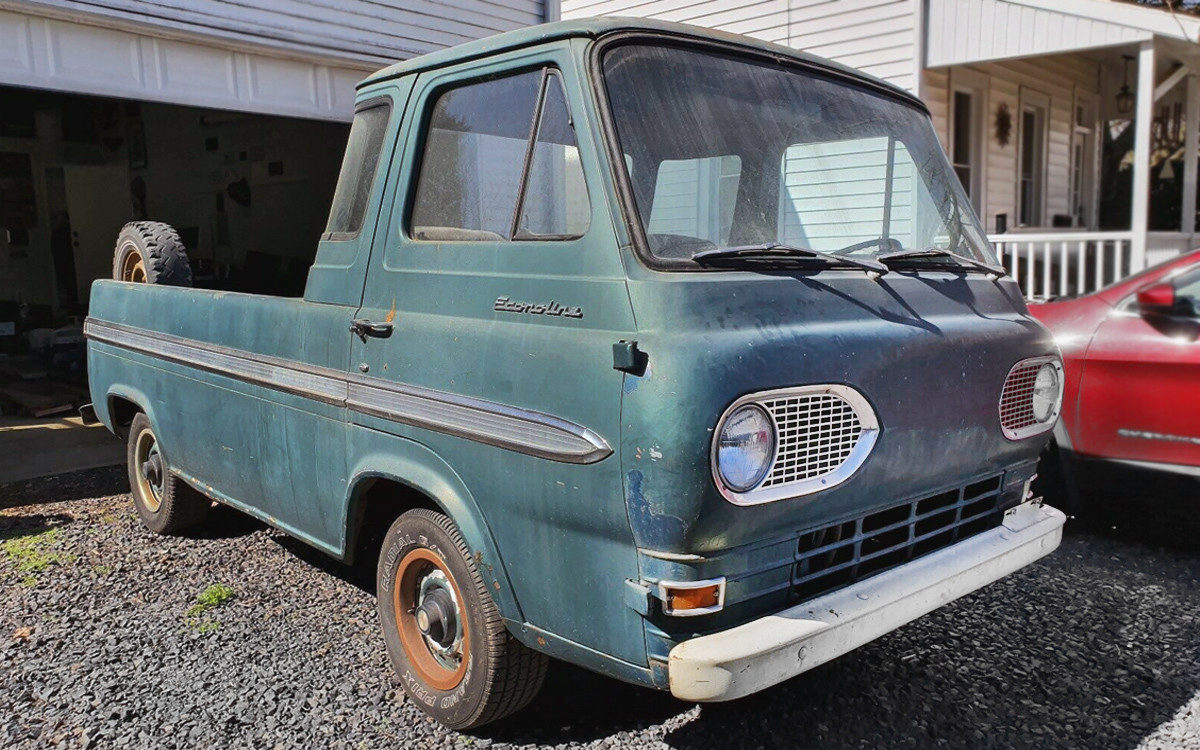The image features a charming, vintage Econoline pickup truck, which appears to be a modified van with its back portion converted into a truck bed. The vehicle is an aged teal-turquoise hue, though the paint is worn and marked by rust and discoloration. Its headlights are small, round, and paired with a distinctive grill, while a long chrome stripe decorates the side. The wheels are mismatched, reminiscent of spare donuts used in emergencies, and there is a tire visible in the truck bed. The truck is parked on a pebble-covered ground with patches of grass or moss, right in front of a garage with a slightly open door. Nearby, partially seen, is a vintage red car, showing only part of its door and side mirror. Both vehicles are set against the backdrop of a white house with a porch and white railing, adding to the nostalgic atmosphere of the scene.